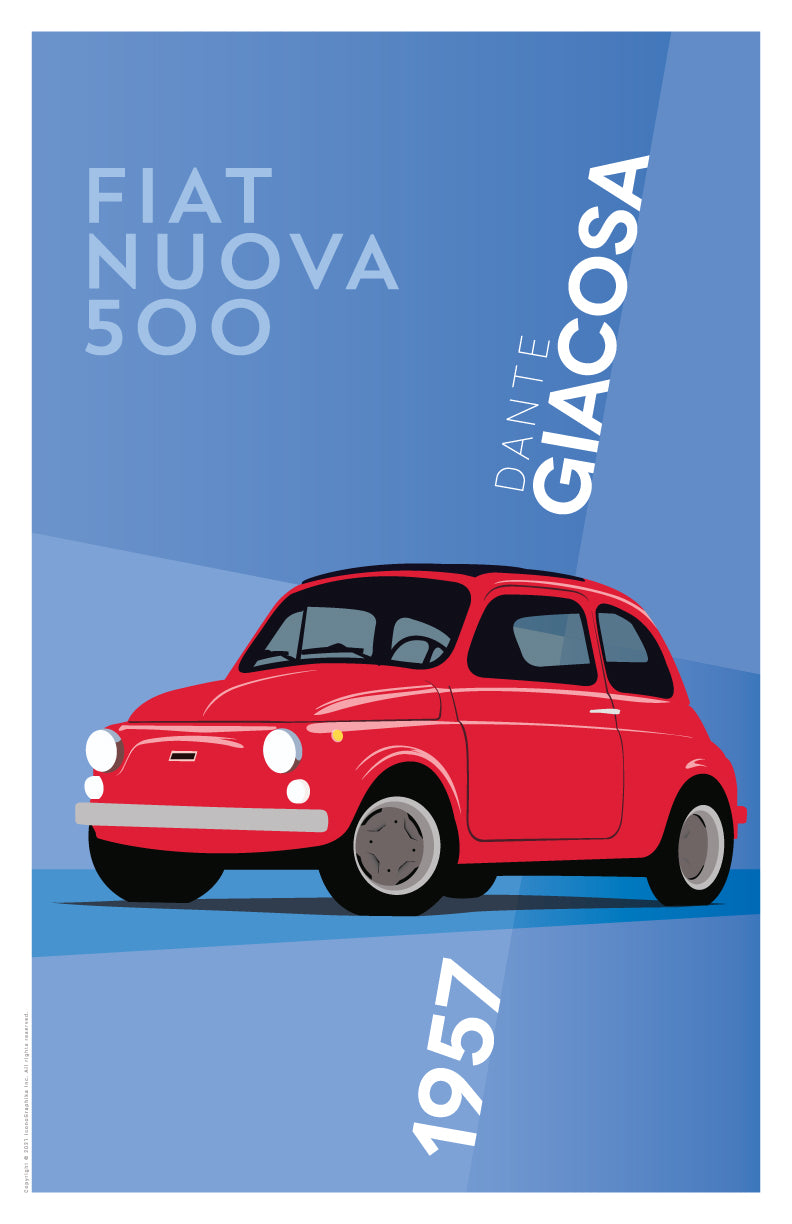The image appears to be a computer-generated advertisement for a vintage car model, styled with Pixar-like colors and design. The background features two shades of blue, setting a vibrant yet retro tone. In the top left corner, the text reads "Fiat Nuova 500" in a lighter blue hue, accentuating the brand and model. The top right corner has white, sideways text stating "Dante Giacosa." 

Dominating the middle of the image is an animated red Fiat Nuova 500 car with a black interior. The car showcases a detailed design, including a silver front bumper, four white headlights, and a sunroof. Despite seeing only one door, it's evident that it's a two-door car. It rides on four black tires with silver rims.

Below the car, continuing the slanted text style, the year "1957" is displayed in white, anchoring the car in its historic context. The overall composition emphasizes clarity and nostalgia, making it a striking modern homage to a classic vehicle.